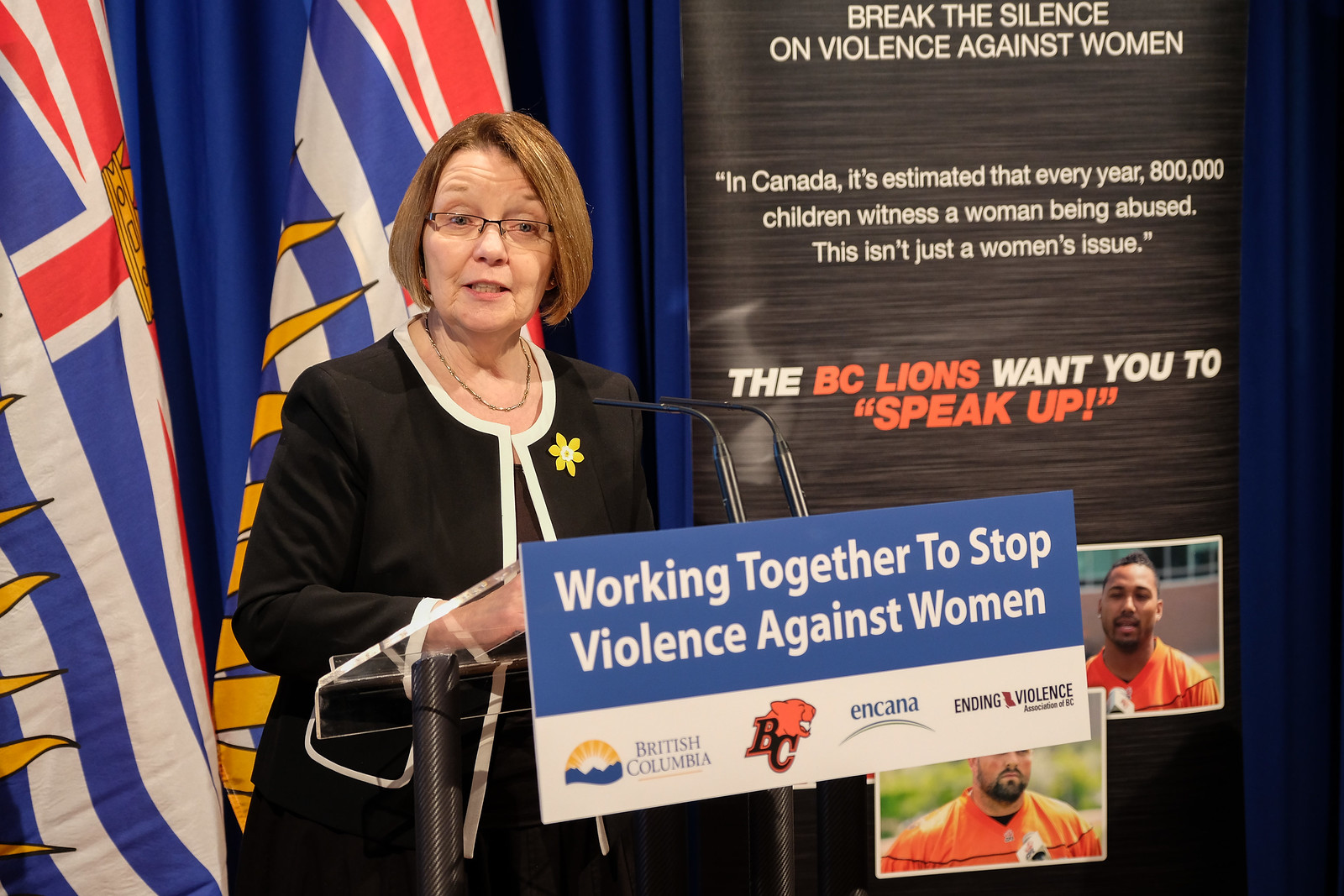A woman with short, slightly reddish-brown hair and glasses is standing slightly left of center at a podium during a conference or rally. She wears a black jacket with white lines around the collar and a yellow flower pin on her left lapel. The podium has microphones angled towards her and a sign in front that reads "Working Together to Stop Violence Against Women," along with emblems for British Columbia, Encana, and an unreadable third sponsor. Behind her is a large banner with text that states, "Break the Silence on Violence Against Women" and includes a call to action from the BC Lions, a Canadian football team. Additional text on the banner highlights that in Canada, every year, 800,000 children witness a woman being abused, emphasizing that this issue affects everyone. The backdrop features flags, curtains, and images of BC Lions members, adding to the appeal for support from the sports community.